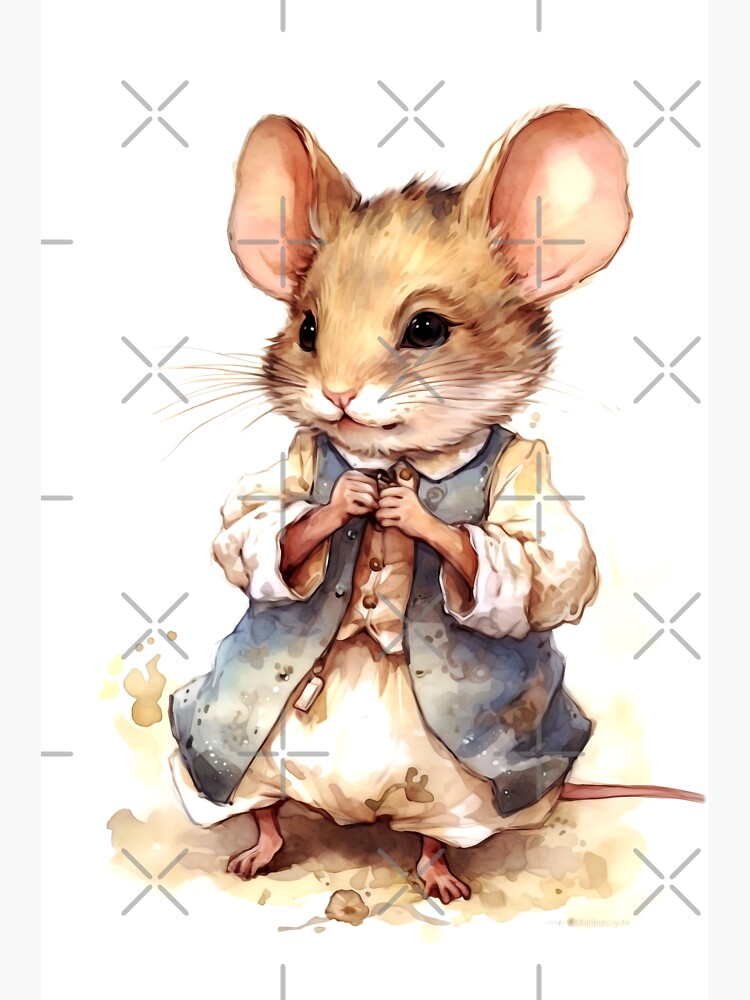The image is a detailed digital or hand-drawn print featuring a small, anthropomorphic mouse standing upright on its hind legs. The mouse has light brown fur with a white mouth and cheek area, and a set of large, pink-inside ears that are almost as big as its head. It has friendly, soft black eyes and a small, pink nose. It is dressed in a white, long-sleeved, loose-fitting shirt that resembles pirate attire, with a large, blue vest that extends to the bottom of its voluminous white pantaloons. The mouse's small pink feet are planted on a muddy surface, matching the dirtied state of its clothing. Its long tail curves out to the left, and the image is overlaid with multiple X-shaped marks, possibly serving as a watermark.